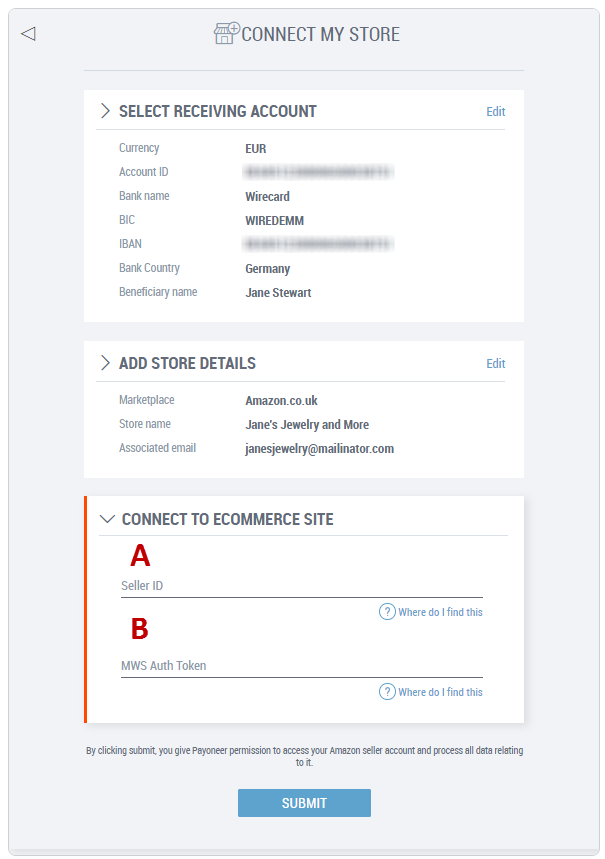Here is the revised caption:

A detailed screenshot of the "Connect My Store" interface captures the steps for linking an Amazon store to an e-commerce platform. The form prompts the user to select a receiving account and requires various banking details including Currency, Account ID, Bank Name, BSC, IBAN, Bank Country, and Beneficiary Name. The interface also includes a section labeled "Add Store Details." Two options are available for e-commerce connection, marked as "Connect to e-commerce site A" and "Connect to e-commerce site B," with a notable red highlight on the left side of one option indicating selection or attention. The background is gray, and a prominent blue "Submit" button is located at the bottom of the screen.